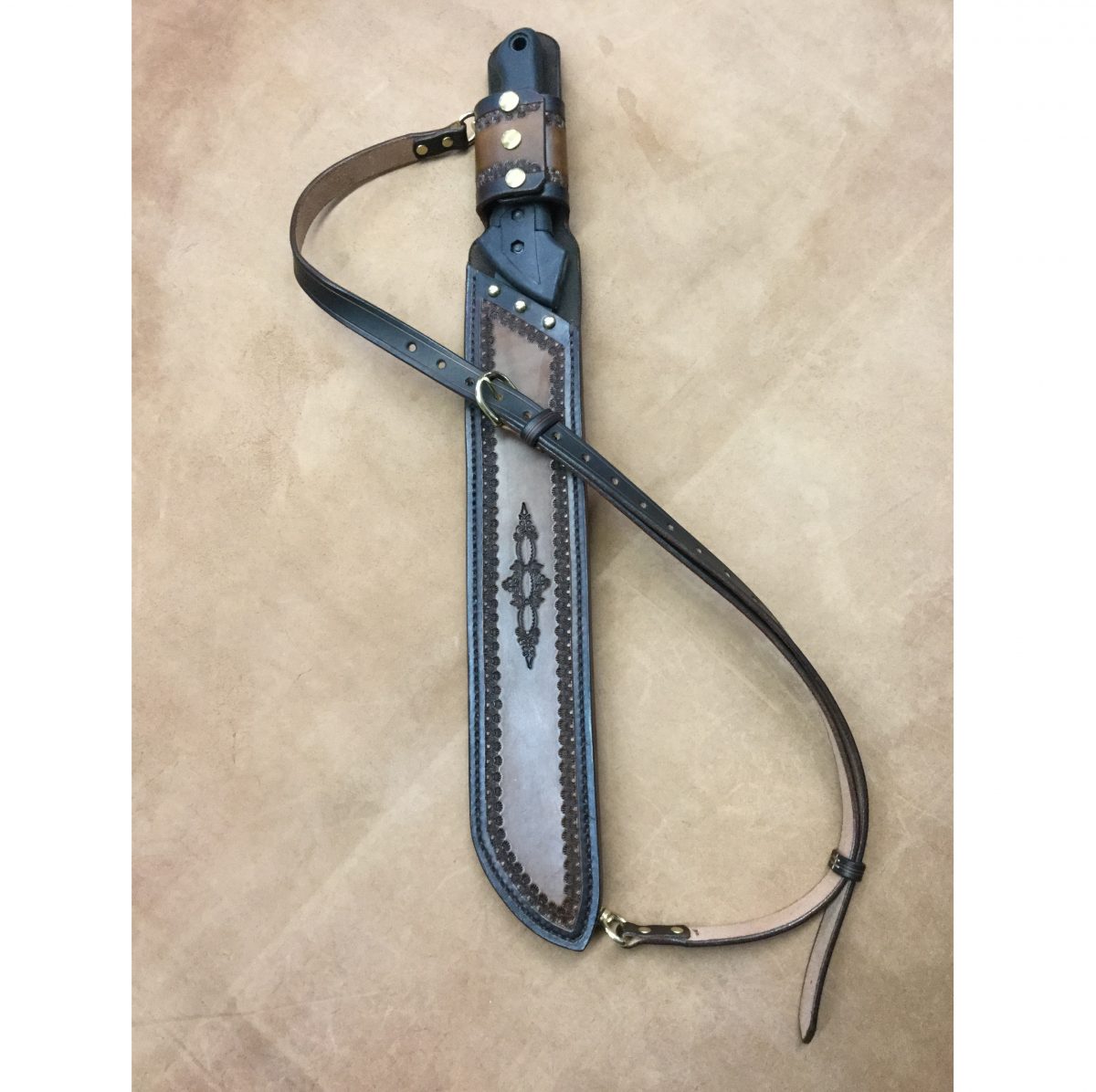The photograph showcases a black knife sheathed in an intricately patterned leather cover, centrally placed against a grainy, light pinkish-brown surface that resembles cut stone. Captured from an overhead perspective, the knife's handle, which appears to be made of dark plastic with a tactical design, is oriented towards the top of the image. The leather sheath features detailed stitching along the edges and includes a decorative strap in the form of an S shape, presumably for attaching the knife to clothing. The overall composition highlights both the rugged, functional aspects of the knife as well as the aesthetic details of its sheath.